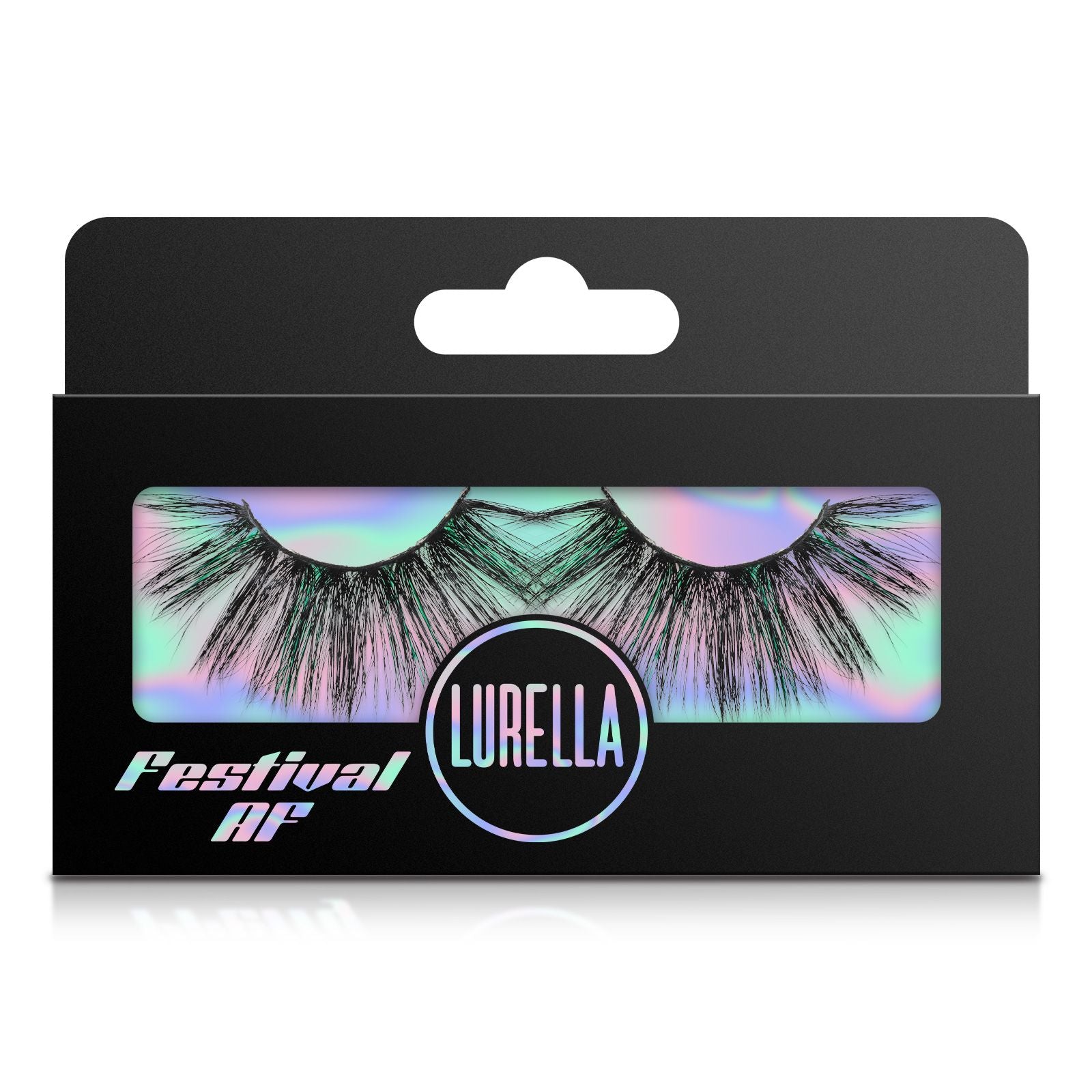The image showcases a close-up of a small, predominantly black box containing a pair of luminous fake eyelashes. The box features a transparent, multicolored plastic window, giving it a rainbow-like appearance and allowing a clear view of the eyelashes inside. At the center of the window is a circular logo with the brand name "Lurella" inscribed in hieroglyphic-style, iridescent colors. Below the logo, on the lower right corner, are the words "Festival AF." The black carton box also includes a traditional punched-out hole at the top for hanging the product on a display rack in a store.